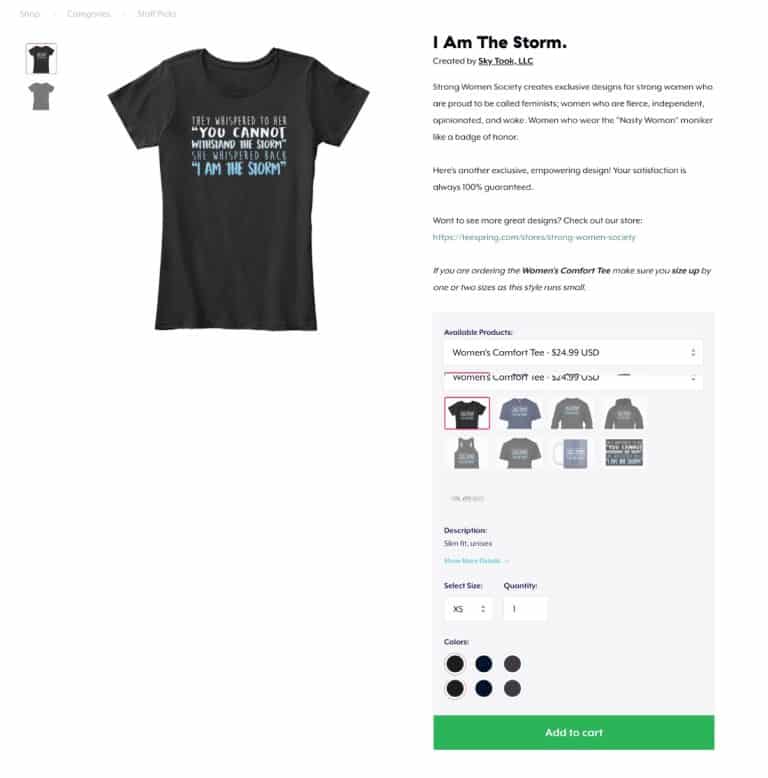The image showcases a product page for a t-shirt sold by the Strong Women Society. The central item is a sleek black t-shirt emblazoned with the empowering tagline, "I am the storm." This tagline is fundamental to the brand's ethos, celebrating strong, feminist women. The t-shirt is displayed from multiple angles, which can be viewed by clicking on the provided thumbnails. 

Below the main image, a detailed description emphasizes the exclusivity and empowering nature of the design. It clearly communicates that customer satisfaction is guaranteed. Notably, it advises customers to size up by one or two sizes when ordering the women's comfort tee, as this style tends to run small.

The bottom section of the image includes a user-friendly order form where customers can select their preferred style, color, size, and quantity of the "I am the storm" t-shirt, priced at $24.99. The process is streamlined with a prominent green "Add to Cart" button that spans the width of the order area, ensuring a smooth shopping experience.